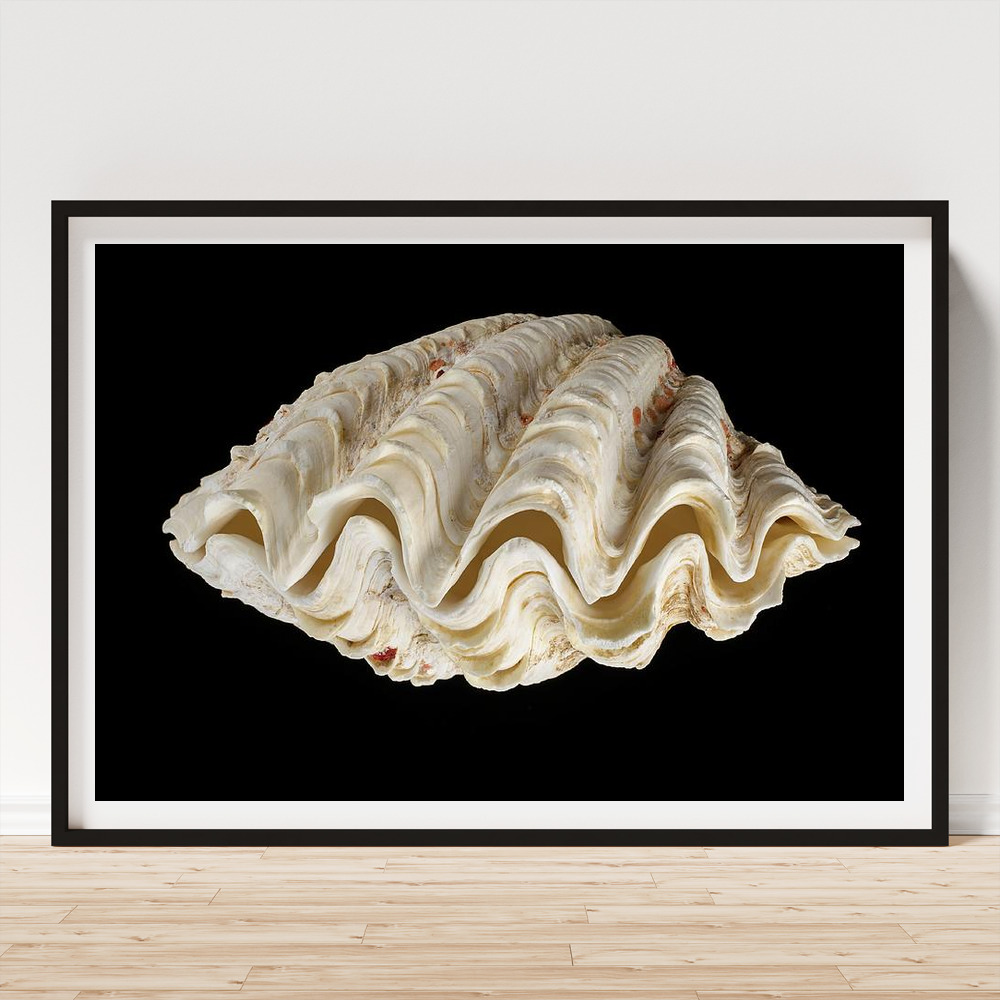A detailed, single descriptive caption for the image would be:

"A large, photorealistic photograph of a clamshell rests on a light wooden floor, leaning against a white wall with subtle gray shadows indicating light from the left. The image is framed in a simple black frame with a white mat. The clamshell, positioned against a solid black background within the photo, appears predominantly off-white with small red and goldish speckles on the top and bottom. While the shell is largely closed, a thin gap reveals its slightly open nature. The shell's surface is characterized by wavy ridges and ripples, giving it a textured, intricate appearance. The overall composition emphasizes the clamshell's large, intricate form, reminiscent of those found at the ocean's depths, powerfully set against the contrasting black background."